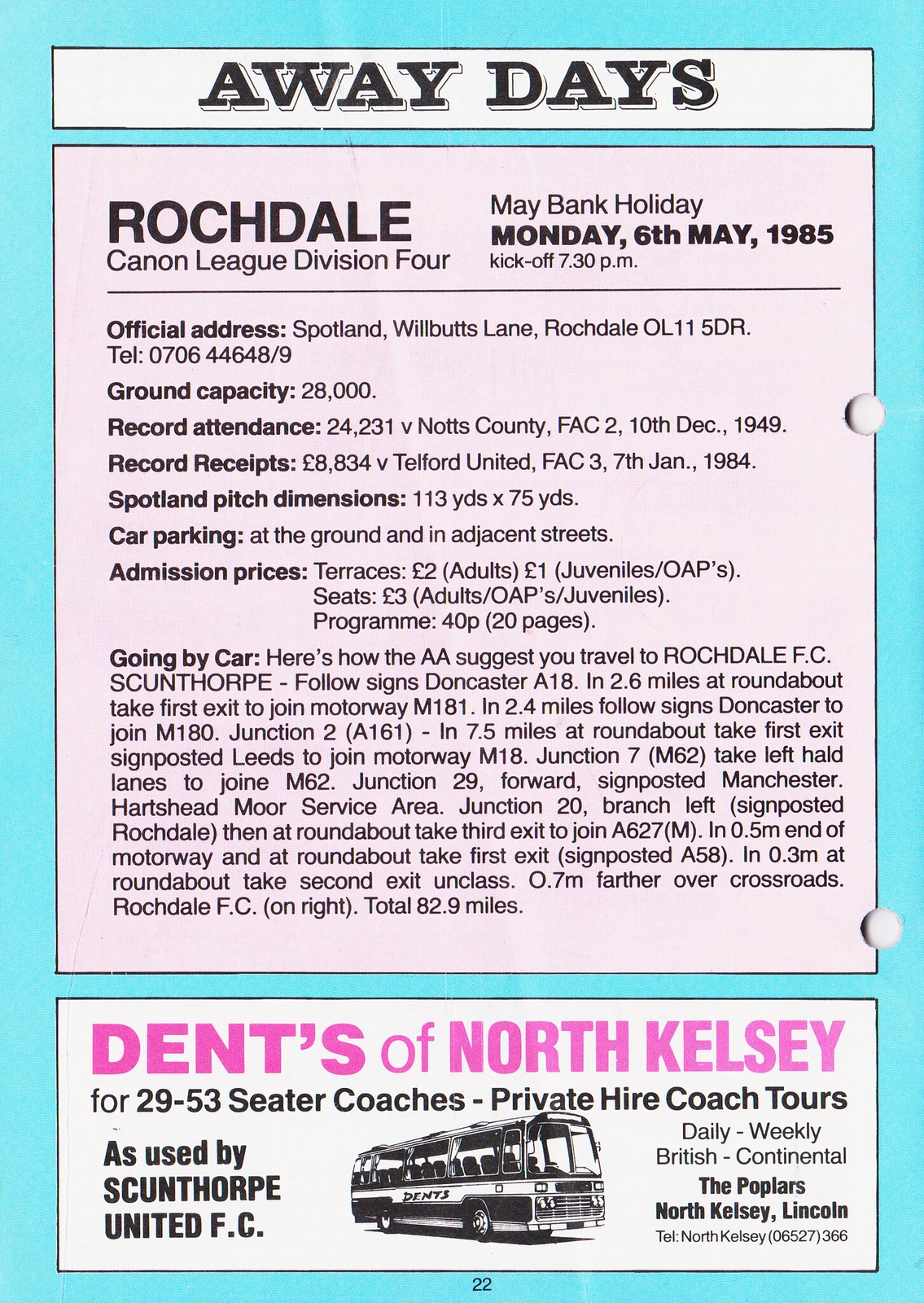The image is a detailed page from a program or poster with a light blue background and three text boxes. The top box has a white background, the middle one features a pink background and contains most of the information, and the bottom box is a white-background advertisement. There are two holes on the right side for placing it in a ring binder. 

The text prominently showcases information for an event titled "Away Days," detailing a Rochdale Cannon League Division 4 match scheduled for Maybank Holiday, Monday, May 6, 1985, with a kickoff at 7:30 pm. The official address for the venue is Spotland-Wilbits Lane, Rochdale, OL-11-5DR, with a contact telephone number 0706-44-648-9. 

Key details include:
- Ground Capacity: 28,000
- Record Attendance: 24,231 (Versus Knotts County, FAC-2, December 10, 1949)
- Record Receipts: 8,834 British Pounds (Versus Telford United, FAC-3, January 7, 1984)
- Pitch Dimensions: 113 yards by 75 yards

For attendees, the program lists various logistics:
- Car Parking: Available at the ground and in adjacent streets
- Admission Prices: Terrace - 2 pounds for adults, 1 pound for juveniles and OAPs; Seats - 3 pounds for adults, juveniles, and OAPs
- Program Cost: 40 pence for 20 pages

Travel instructions provided by the AA suggest a detailed route to the Spotland ground, covering multiple highways and roundabouts, mentioning specifics like Junctions M181, M180, and M18, taking you through motorways and service areas. 

The advertisement at the bottom highlights North Kelsey Coach Tours, offering private hire coaches and tours, used by the Scunthorpe United FC, with contact info: North Kelsey, Lincoln, Telephone 0652736622. 

Overall, this page provides comprehensive information about the match, venue, travel routes, ticket prices, and additional services with a structured and easy-to-follow layout.